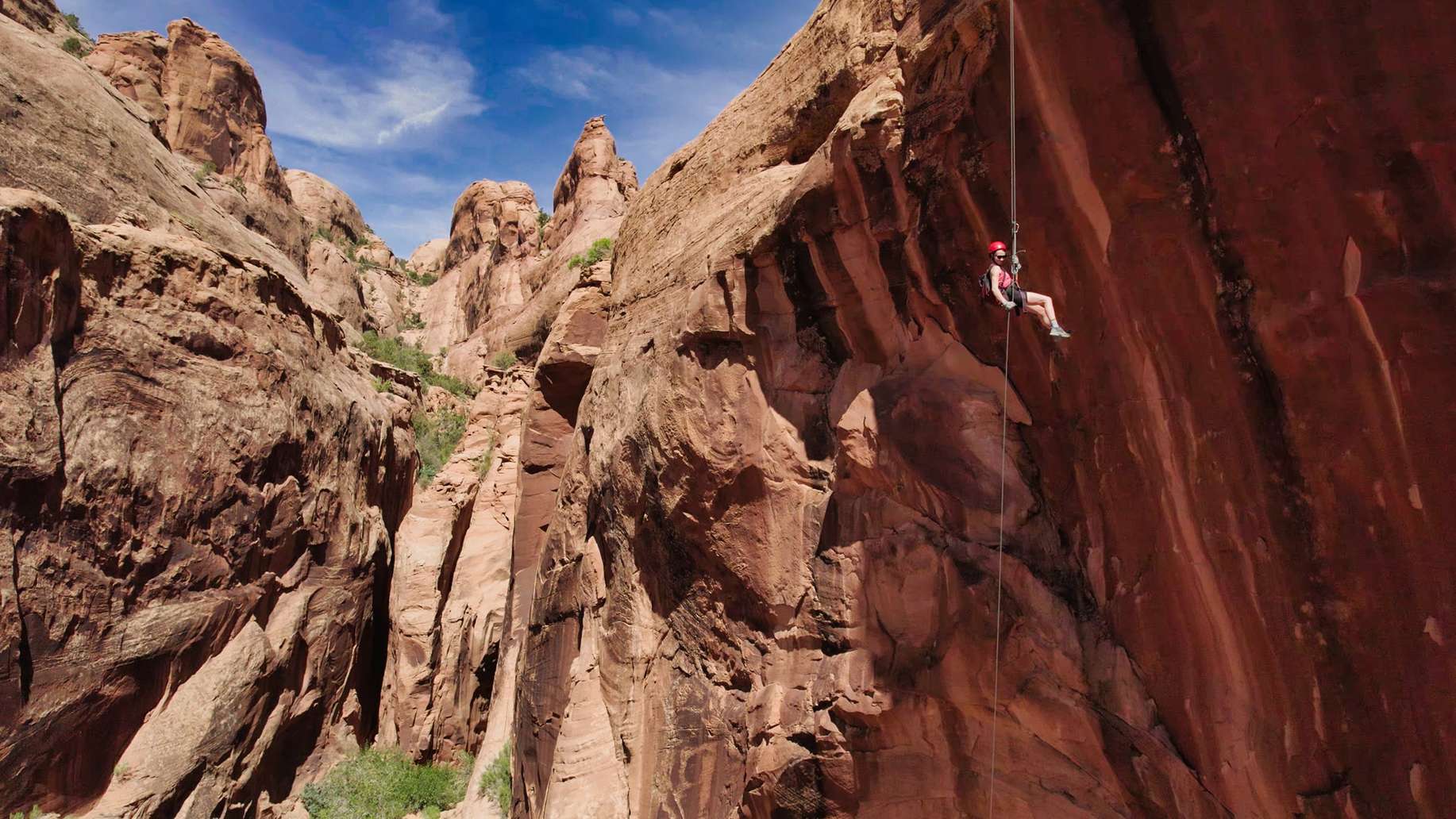The image captures a striking scene of a young woman, approximately 25 to 30 years old, rappelling down a steep, brownish-red cliff in a mountainous desert region, possibly in Utah. The young woman, who appears to be white, is secured by a single rope and is fully equipped with rock climbing gear. She wears a red helmet, black sunglasses, a pink shirt, and athletic shoes, highlighting her adventurous spirit. The cliff, seen from a low vantage point looking up, towers high into a partly overcast yet blue sky, adorned with wispy clouds. The rock face is intermittently adorned with patches of grass and other greenery. This breathtaking and potentially perilous activity underscores the thrill and physical strength required for rock climbing, suggesting the presence of another person capturing this daring moment.